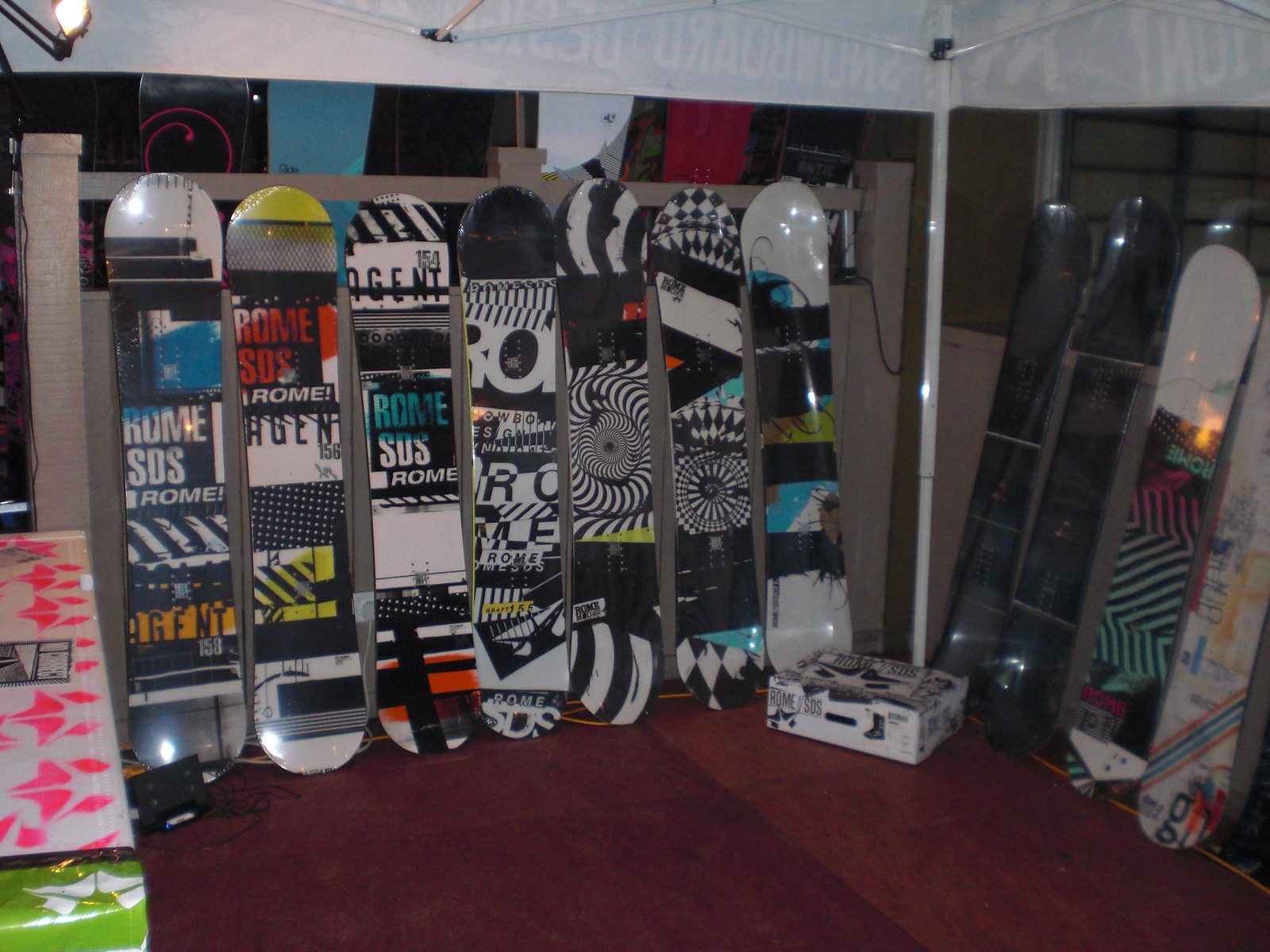The photograph captures multiple snowboards in a dimly lit environment. The snowboards, showcasing a variety of busy designs with vibrant spirals, words, and colors including black, white, red, yellow, blue, and orange, are leaning against a white-colored wall and gray posts. The majority of the boards are wrapped in their original packaging, suggesting they are brand new and ready to be sold. Some of the boards feature distinct wordings such as "Rome SOS," "Rome SDS," and "agent." A total of seven snowboards are prominently displayed at the center, while four additional snowboards are seen hanging nearby. These boards rest on a floor that varies in description—some parts appear to be dark hardwood, while others have a fuzzy red and orange texture. An overhead light in the top left corner illuminates the scene, adding a warm glow. In the lower left corner, there's another snowboard colored with white, pink, and green hues. The top part of the image features a white section, and a white cable and a white box with black text and imagery are visible on the floor along the right side. The overall setting suggests this scene could either be inside a storage unit or outside, sheltered under a white tarp, amidst the night.